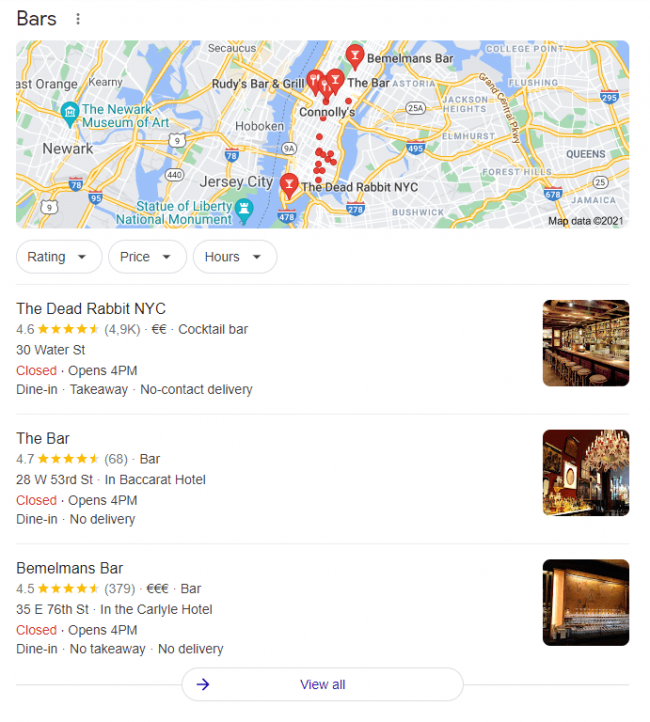A detailed caption for the image could be:

"A screenshot taken on a phone, tablet, or computer displaying a search for bars near Jersey City, visible on a map adorned with red pinpoints. This map showcases landmarks such as the Statue of Liberty National Monument, waterways, and roads. Notable search results feature icons depicting either a cup, representing alcoholic drinks, or a fork and spoon for dining. Below the map, a drop-down menu offers filtration options for rating, price, and hours. Two highlighted establishments are 'The Dead Rabbit NYC' and 'The Bellman's Hand,' each accompanied by star ratings and interior photos on the right side. Both bars seem to have garnered positive reviews."